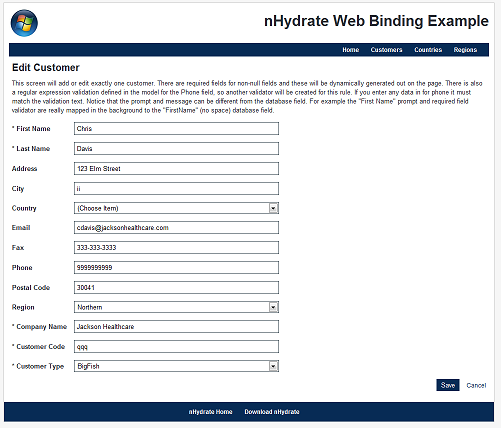The image depicts a screenshot of a website with a clean, white background. In the top left corner, there is a blue circle with the Microsoft logo inside it, consisting of four small, diagonal squares that form a larger square. The colors of these squares are red (top-left), green (top-right), blue (bottom-left), and yellow (bottom-right).

On the far right side, there is text in a blue font that reads "NHydrate," with the "N" and "H" capitalized. Beneath this, the site description "web, binding example" is written in smaller, mixed-case blue font. Just below, there is a dark blue banner featuring white font links for navigation labeled "Home," "Customers," "Contacts," and "Reports."

Under this banner, towards the left side, there is a bold blue header reading "Edit Customer," indicating that this screen is used to hold or edit information for a single customer. Following this, there is an explanation about the required fields for the form below.

The form consists of multiple text input boxes with consistent height and a blue font. Each input field label has an italicized asterisk prefixing the text, indicating that these fields are mandatory. The labels are: "First Name," "Last Name," "Address," "City," "Country," "Email," "Fax," "Phone," "Postal Code," "Region," "Company Name," "Customer Code," and "Customer Type."